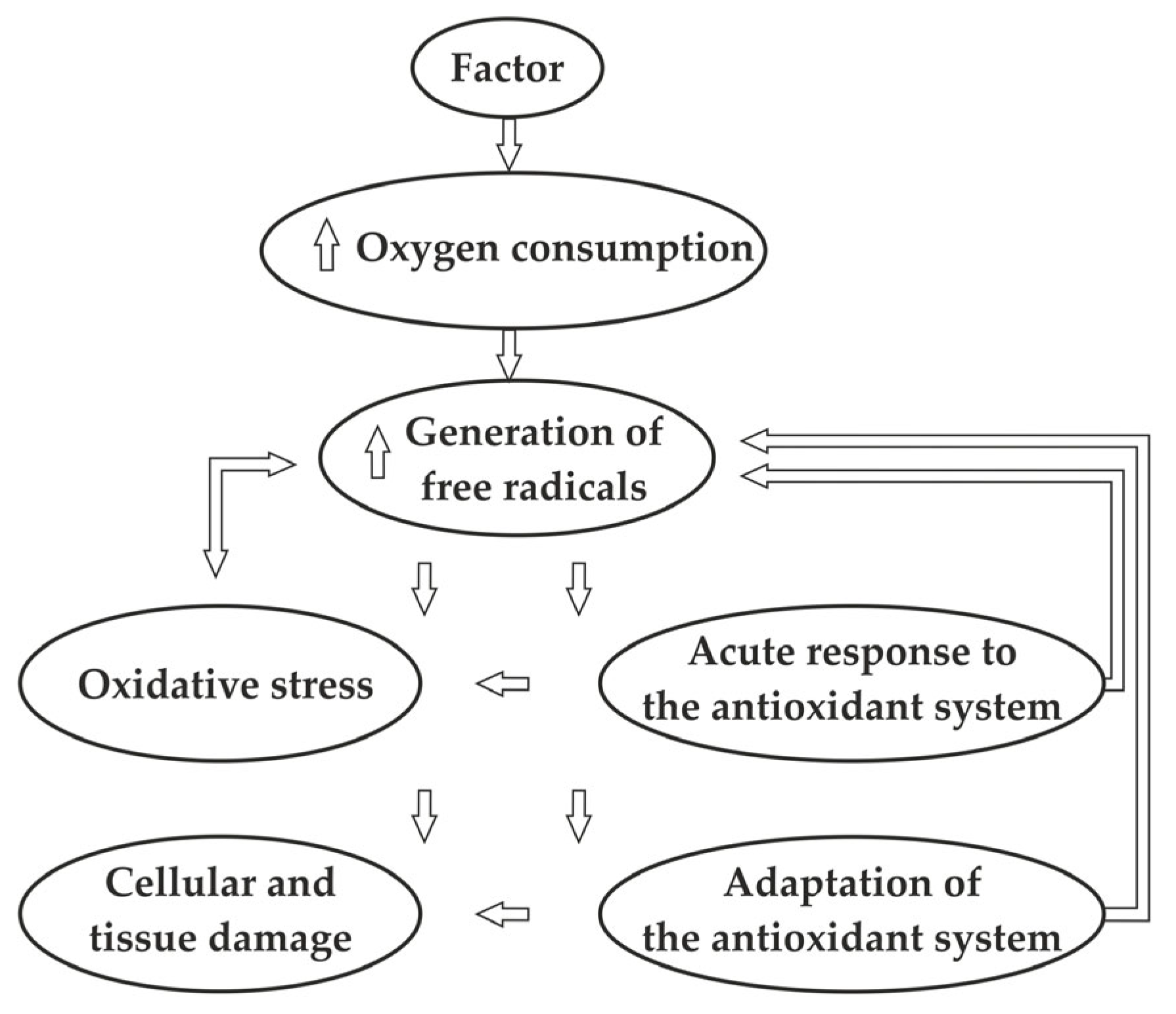The image is a detailed black-and-white flowchart presented on a white background, with black text inside horizontally oriented ovals, outlined in black. At the top center, the word "FACTOR" is circled, followed by a downward arrow leading to "OXYGEN CONSUMPTION." An internal arrow within this oval points back up to "FACTOR," while an external arrow points down to "GENERATION OF FREE RADICALS." This circled term contains an internal upward arrow pointing back to "OXYGEN CONSUMPTION" and two external downward arrows. Continuing downward, this flow is connected to four more circled terms: on the left is "OXIDATIVE STRESS," on the right is "ACUTE RESPONSE TO ANTIOXIDANT SYSTEM." At the bottom left is "CELLULAR AND TISSUE DAMAGE," and at the bottom right is "ADAPTATION OF ANTIOXIDANT SYSTEM." Various arrows connect these terms back to previous stages in the flowchart, illustrating a complex interplay and feedback loop between the different components.